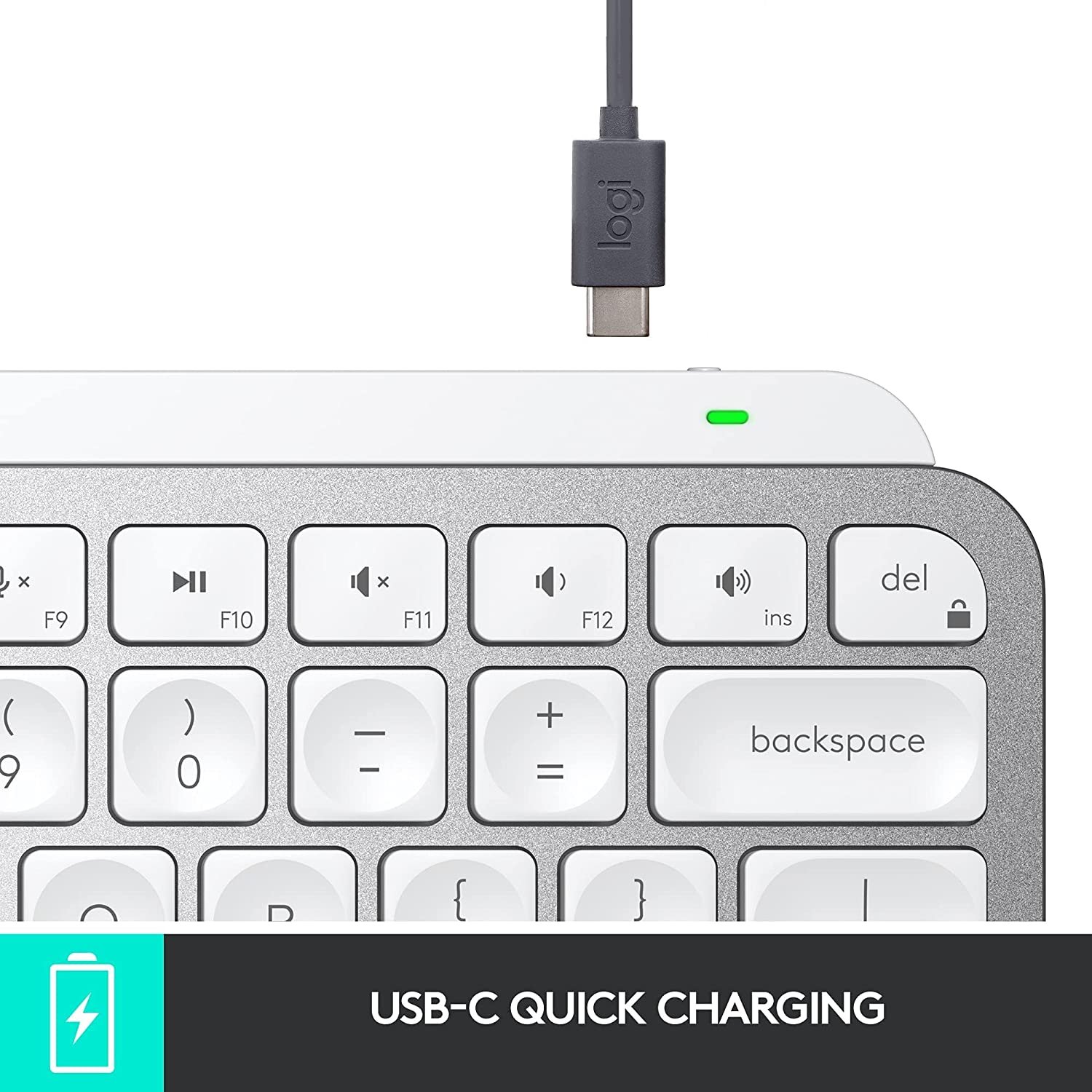The image is a close-up of the top right-hand corner of a silver keyboard, showcasing a variety of keys and a charging setup. Visible keys include F9 through F12, the Insert and Delete keys, the numbered keys 9 and 0, the dash and plus keys, and the Backspace key. Additionally, parts of five keys below are partially visible. A black charging cord, which has a silver port and a black base labeled "Logi," is positioned over the keyboard. In the background, there's a long, oval-shaped green light glowing. At the bottom right corner of the image, there is a black banner that reads "USB-C quick charging" in white text. To the left of this banner is a turquoise square featuring a white battery symbol with a lightning bolt on it. This appears to be a professional, possibly stock, image promoting the keyboard's USB-C quick charging feature.